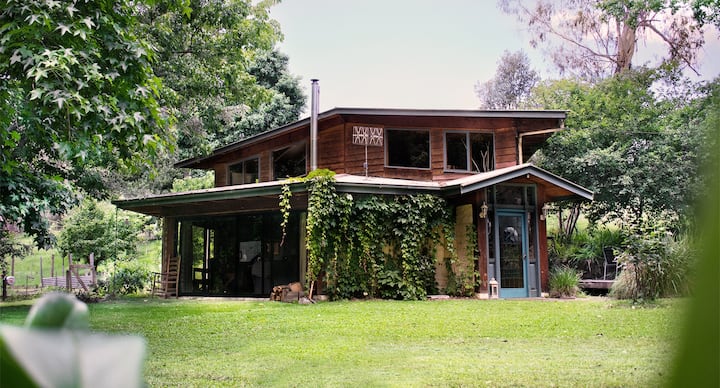The photograph presents a clear, detailed outdoor view of a charming, simple two-story house set amidst a well-maintained green lawn and surrounded by numerous trees. The house features a blue door on the front and is predominantly a brownish or reddish rust color. Ivy, or possibly other climbing plants, decorates the facade up to the roof level on the left side. There are two windows visible on both the upper front and side.

A flat-looking roof, as perceived from the angle, covers the home. The roof extends to form a small portico over the front door, creating a subtle elevation variation. There is a rocker situated under an awning or a big doorway at the back, adding to the cozy, country charm of the home. 

Notably, a pipe sticks out from the corner of the house, and there is a ladder leaning against a tree to the left. The sky above is gray, though in some descriptions it appears bright, suggesting natural light conditions.

In the background, the greenery includes tall, mature trees, which provide a picturesque frame to the house. Despite no visible presence of people, cars, or pets, the image radiates a serene, rural ambiance.